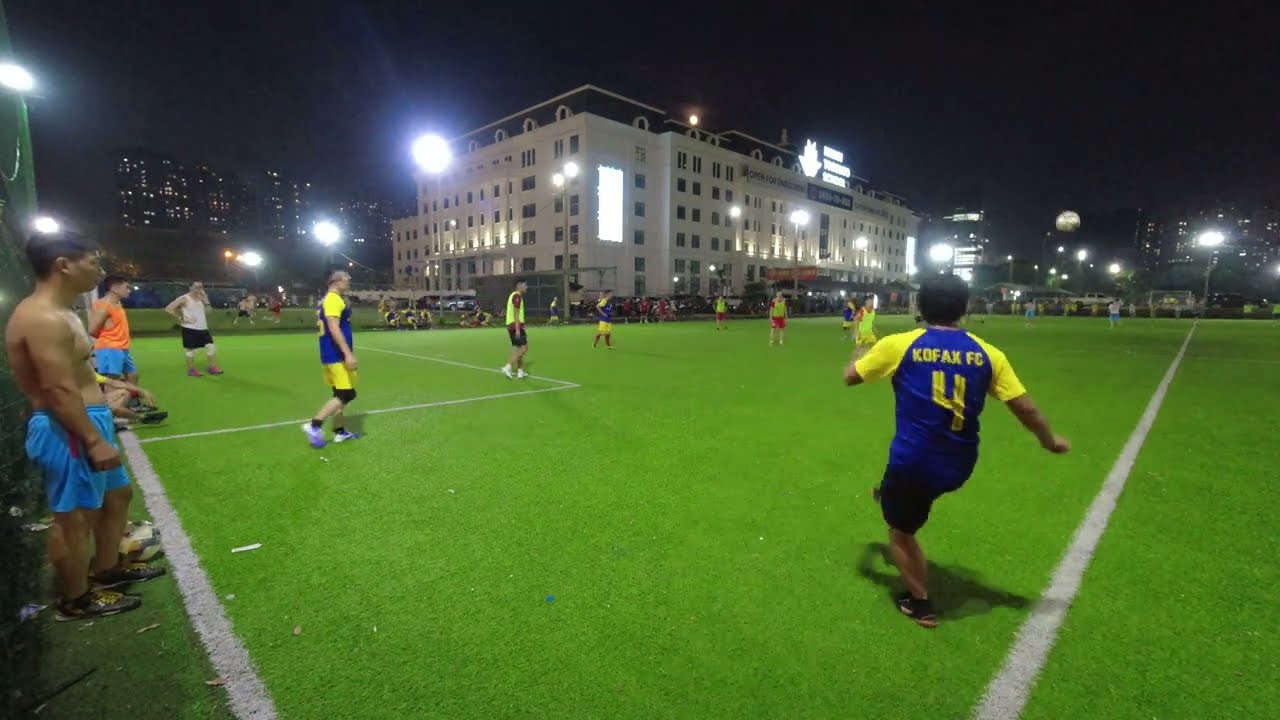In this nighttime soccer scene, a group of about 6 to 7 players is actively engaged in a game on a lush, light green field marked with boundary lines. The field, possibly made of grass or artificial turf, is brightly illuminated by tall floodlights. The main player in focus wears a blue and yellow jersey with the number 4 and the text "COFAX FC" on his back. To his left, more players in blue and yellow, as well as red and green jerseys, are scattered across the field. One individual, shirtless and possibly resting, stands on the left side, alongside another person in an orange tank top and blue shorts. In the middle of the field, a figure—likely the referee—wearing a light green vest and black pants, can be seen orchestrating the game.

In the background, a large building, possibly a hotel resort or hospital, stands prominently with its many lit windows and distinct rectangular illumination on one side, casting additional light onto the field. Surrounding the field on the left and right are more buildings, their details obscured by the darkness but hinted at by scattered lights. The sky overhead is a deep, unbroken blue, devoid of any visible moon or stars. Tucked away behind the buildings on the right are some parked cars and additional lights, adding further context to the urban setting. Spectators, including a shirtless man and another person with an orange shirt, watch the game from a grassy area, blending into the lively and dynamic atmosphere of the night-time sporting event.